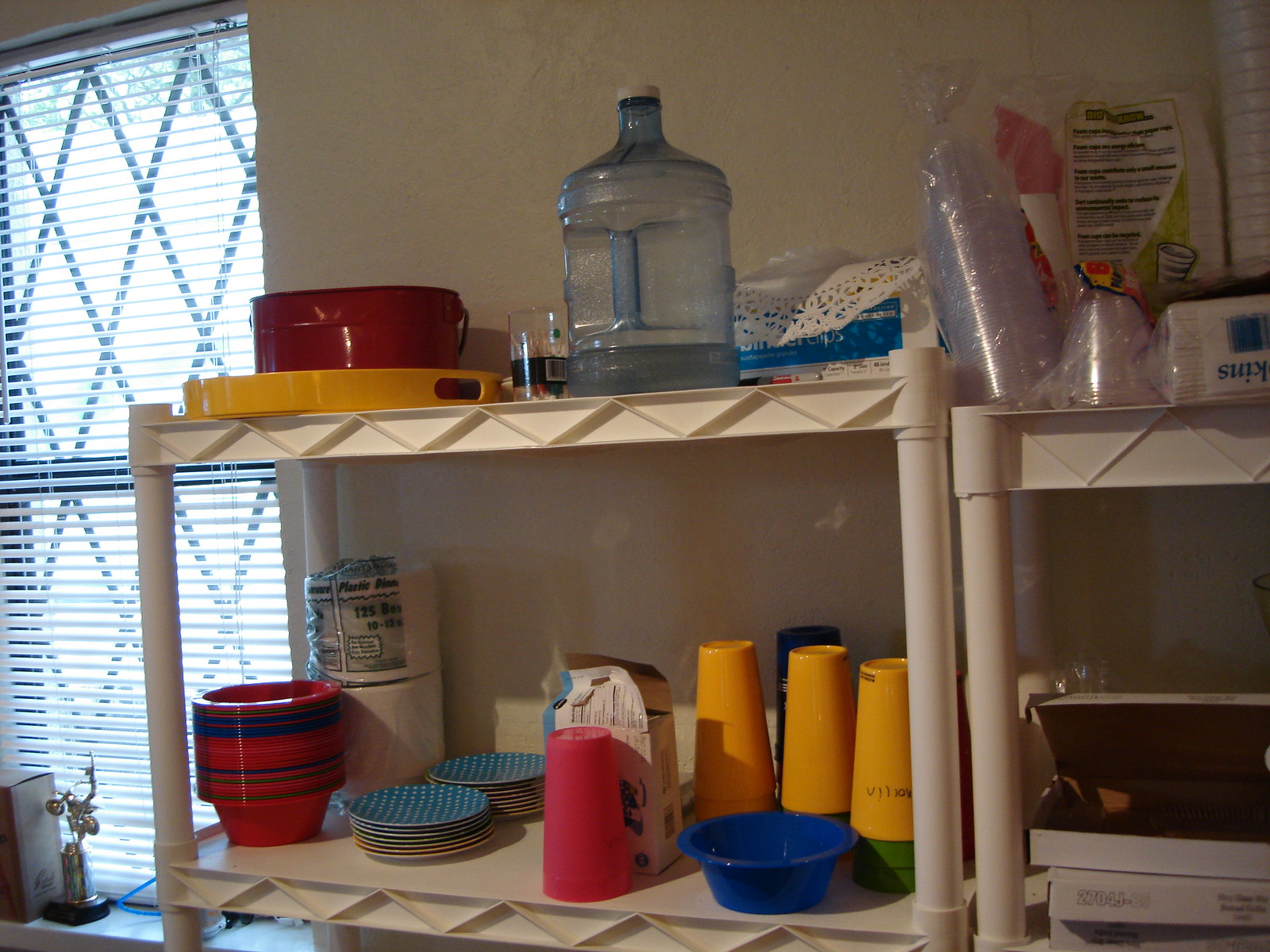The photo captures a well-stocked kitchen, with a myriad of details adding to its cozy ambiance. On the left side of the image, there is a narrow rectangular window adorned with blinds, letting in the natural light. Sitting on the windowsill is a decorative ornament, seemingly an award or commemorative piece, next to a book. Beyond the window, there is a diamond-shaped grille offering a glimpse of the outside.

Inside the room, the notable feature is the shelving unit with two white rails. The top shelf hosts a variety of items including a yellow tray containing a red bowl or bucket, a glass wrapped in black, a large clear bottle with a white lid, and a package with a blue and white design.

On the lower shelf, a bag of plastic cups, a package of toilet paper with a yellow-green hue, and an open white pizza box among three pizza boxes can be seen. Additionally, there are stacked cups – yellow on top of green – and a collection of kiddie bowls in blue, red, and green. Further details include a pink cup, a white box, blue plates with white dots, and more plastic ware meticulously arranged. The shelves are efficiently packed, with visible toilet paper at the back.